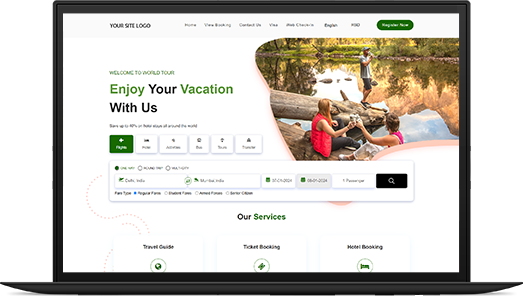The image features a laptop screen displaying the homepage of the "WorldTour" website. Prominently positioned at the top of the webpage is the site logo, followed by navigation options including "Home," "View Booking," "Contact Us," and a language selector set to "English." A highlighted "Register Now" button invites new users to join. The welcoming message reads, "Welcome to WorldTour. Enjoy your vacation with us." The menu offers several options: "Travel Guide," "Ticket Booking," "Model Booking," and "Our Services." The repeated phrase "Welcome to WorldTour" underscores the site's inviting and user-friendly atmosphere.